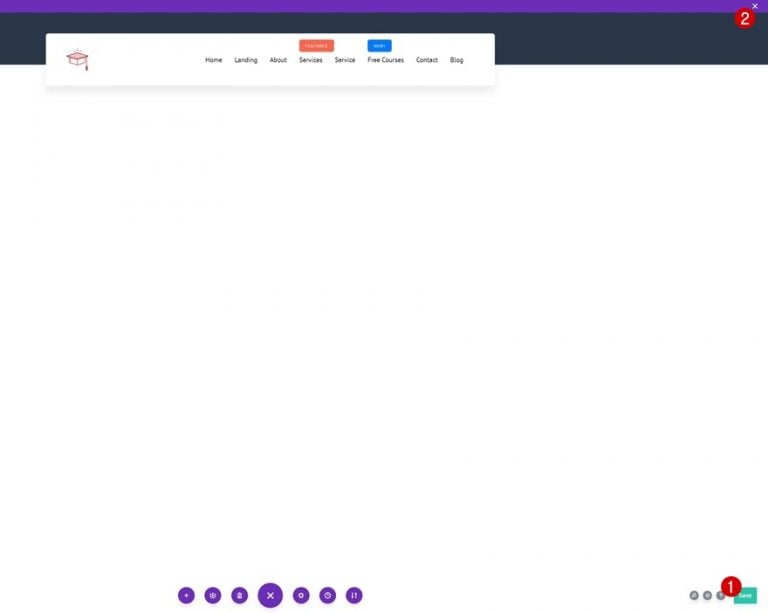Here is a clean and detailed caption for the described website image:

---

The website features a gradient design along the upper edge, transitioning from purple at the top to black below. On the left side of the black section, a white rectangle floats prominently, almost reaching the edge. Within this rectangle, black text displays navigation links: "Home," "Landing," "About," "Services," "Service," "Free Courses," "Contact," and "Blog." Additionally, there is a red button and a blue button, although the text on these buttons is too blurry to read.

The majority of the page is dominated by a white background. At the very bottom, a series of small purple circles are aligned: three on the left, a larger central circle, and three on the right. The large central circle features a white X, while among the smaller circles, the leftmost one shows a plus sign, one might resemble a trash can, another shows a clock icon, and another looks like a download/upload button.

On the right side of the page, three gray circles with white interiors can be observed. There appears to be a green button labeled "Save," but the text is uncertain. Two red circles with numbers are present: the first one with the number "1" on the green "Save" button in the bottom right corner, and the second one with the number "2" in the upper right corner near a white X, which likely serves as a close button for the page or site.